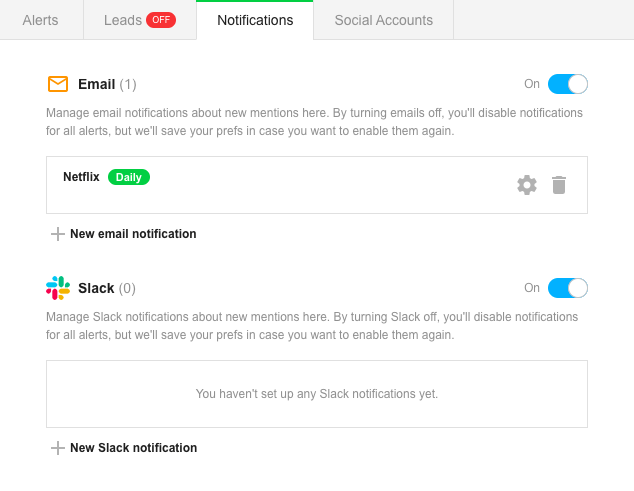The interface displays several tabs at the top, with the first tab highlighted in red, labeled "Alerts." Adjacent to it are tabs for "Notifications," "Social Accounts," and a selection currently on "Notifications." The interface features a green line at the top against a white background, while other sections are predominantly grey with grey text, except for the active tab which has black text. 

Beneath the tabs, within the "Notifications" section, there is text indicating: "Email (1)," followed by the instruction, "Manage email notifications about new mentions here. By turning emails off, you'll disable notifications for all alerts. We will save your preferences in case you want to enable them again." This notification option is currently toggled on, indicated by a blue switch.

Directly below, there is a section titled "Netflix Daily," displayed with a green background and white text. To the right of this section, there are icons for settings and a trash can.

Further down, under the heading "New Email Notifications," there is an entry for "Slack (0)", accompanied by the text, "Manage your Slack notifications about new mentions here. By turning off Slack, you'll disable notifications for all alerts. We will save your preferences in case you want to enable them again." This setting is also toggled on and it is blue in color. A note beneath states, "You haven't set up any Slack notifications yet."

On the left side of this section, there is a "New Slack Notifications" link featuring a plus sign. The interface uses a color scheme that includes grey, red, green, blue, yellow, orange, and black.